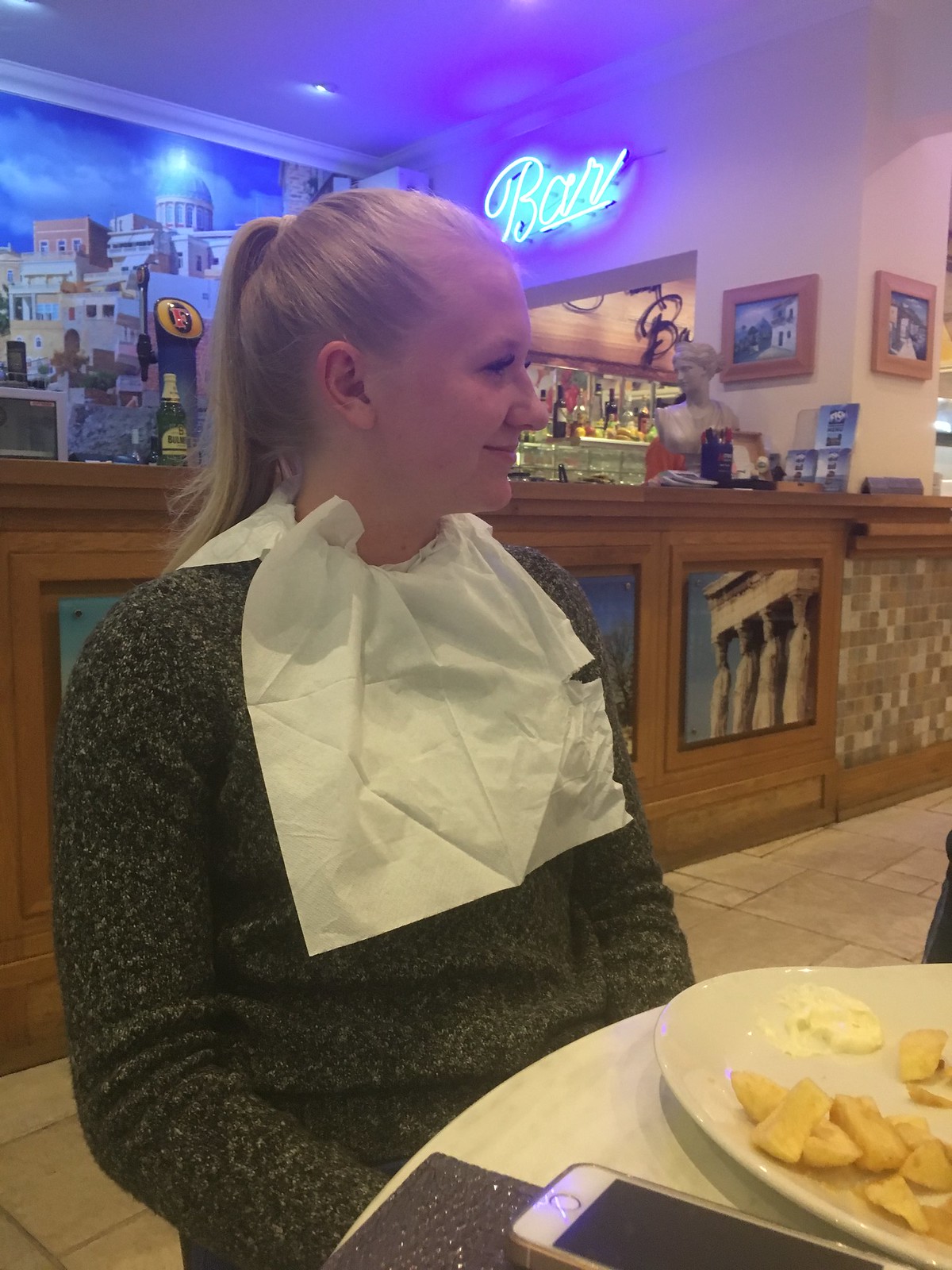In this indoor restaurant setting, a young blonde woman with light skin and her hair pulled back in a ponytail sits at a round, white table. She is dressed in a long-sleeved charcoal gray sweater adorned with white speckles and has a white napkin tucked into her collar like a bib. She faces to the left, seemingly engaged in conversation. The table holds a white plate with thick, golden French fries and a dollop of white sauce. An iPhone with a bronze case lies at the lower right corner of the table. Behind her, a bar crafted from brown wood stands out, with its front transitioning to stone or tile in shades of tan. The back wall of the bar is decorated with photographs of Roman buildings and is illuminated by a blue neon light spelling out "bar," casting a slightly purple hue over the area. The ceiling above features a blue light that integrates into the overall ambiance.